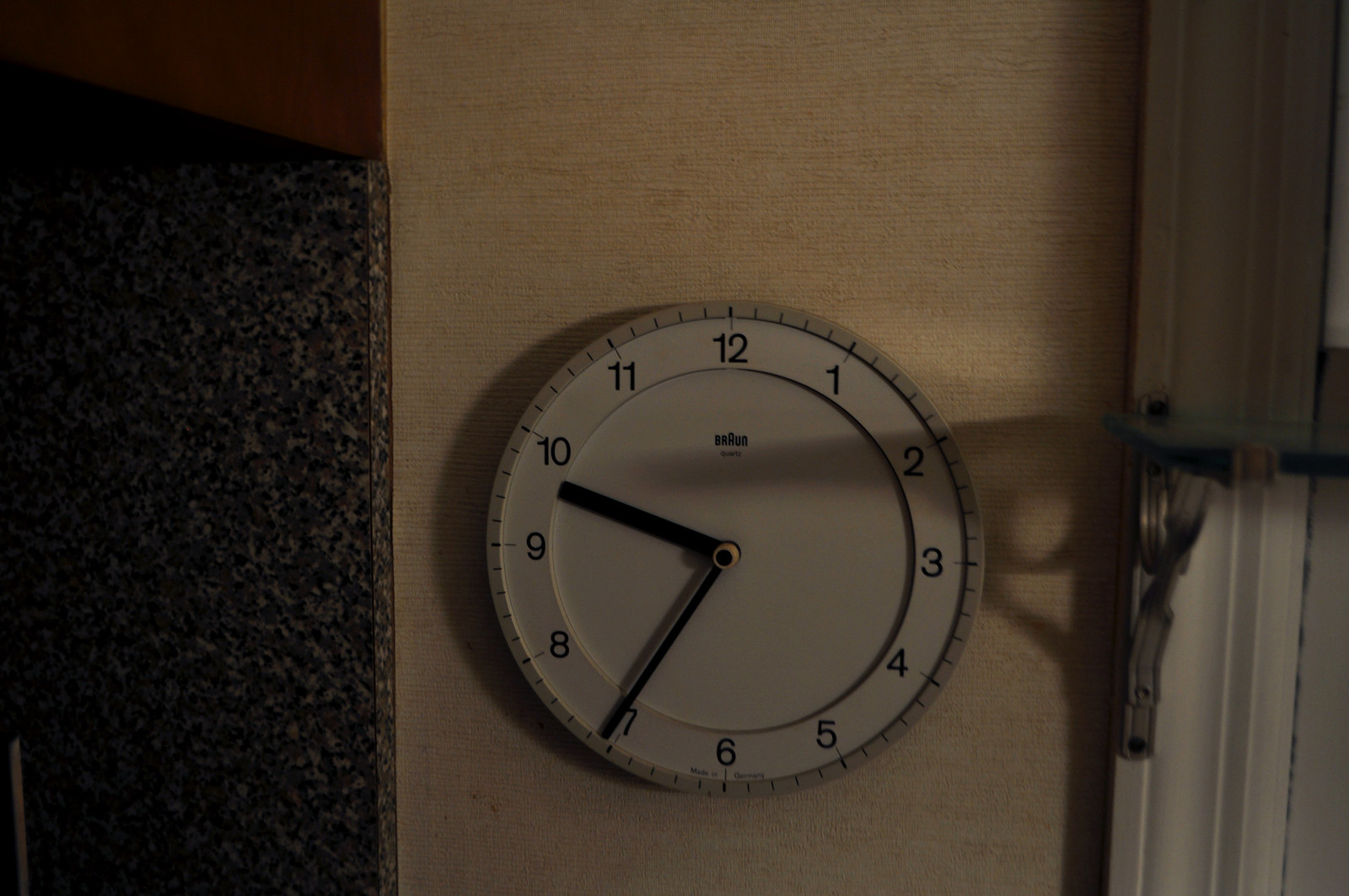This color photograph captures a clock mounted on an oatmeal-brown wall in a dimly lit room with low exposure. The clock, which reads 9:35, has a white face adorned with black numerals and the brand name "Braun" positioned just below the 12. The hour hand is just before the 10, and the minute hand points to the 7. Surrounding the white clock face is a circumference of light brown ridges. 

To the right of the clock, there's a grey shelving unit, possibly holding up a glass shelf, resting on a white door or window frame. This area also receives some light filtering through the windows. On the left side of the wall, there is a dark black and white speckled marble piece, which appears to be either real or faux. Just above this marble piece, the wall transitions into a dark red hue. The scattered light and the shadows cast by elements on the wall add depth and contrast, enhancing the overall atmospheric composition of the image.